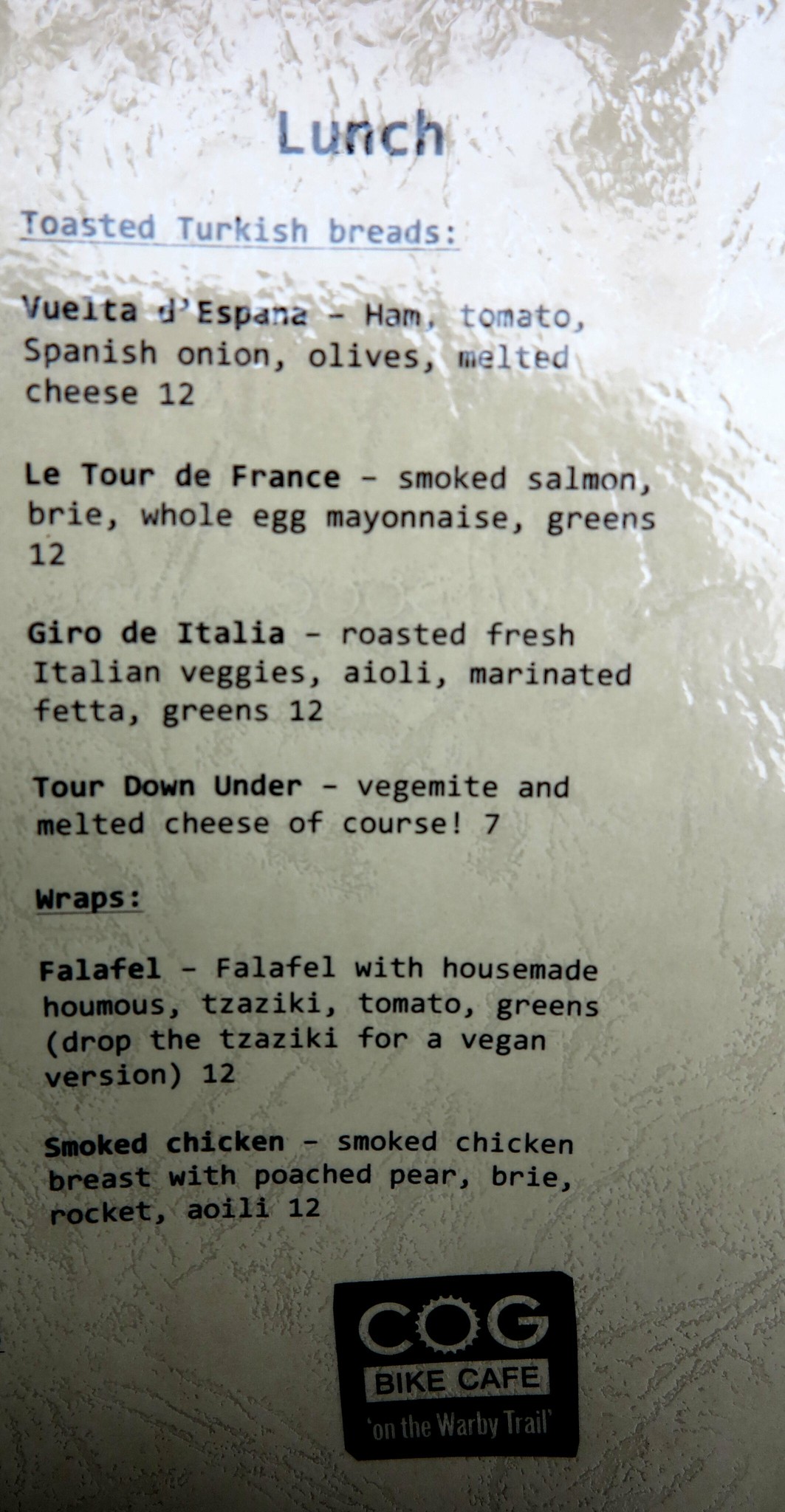The image depicts a sleek and shiny, possibly laminated, lunch menu from the Cog Bike Cafe, located on the Warby Trail. The color scheme of the menu is primarily black, white, and gray. At the very top, in bold black letters, it reads "Lunch," followed by "Toasted Turkish Breads:" underneath which are listed four gourmet options. The "Vuelta de España" features ham, tomato, Spanish onion, olives, and melted cheese for $12; the "Le Tour de France" includes smoked salmon, brie, whole egg, mayonnaise, and greens for $12; the "Giro d'Italia" offers roasted fresh Italian veggies, aioli, marinated feta, and greens for $12; and the "Tour Down Under" features Vegemite and melted cheese for $7. 

Following this section, there is a line underlined with "Wraps" introducing the next items. The "Falafel wrap" contains falafel with house-made hummus, tzatziki, tomato, and greens, with an option to drop the tzatziki for a vegan version, all for $12. The "Smoked Chicken wrap" includes smoked chicken breast with poached pear, brie, rocket, and aioli, also for $12. At the very bottom of the menu, there is a small black square logo that labels the establishment as Cog Bike Cafe on the Warby Trail.